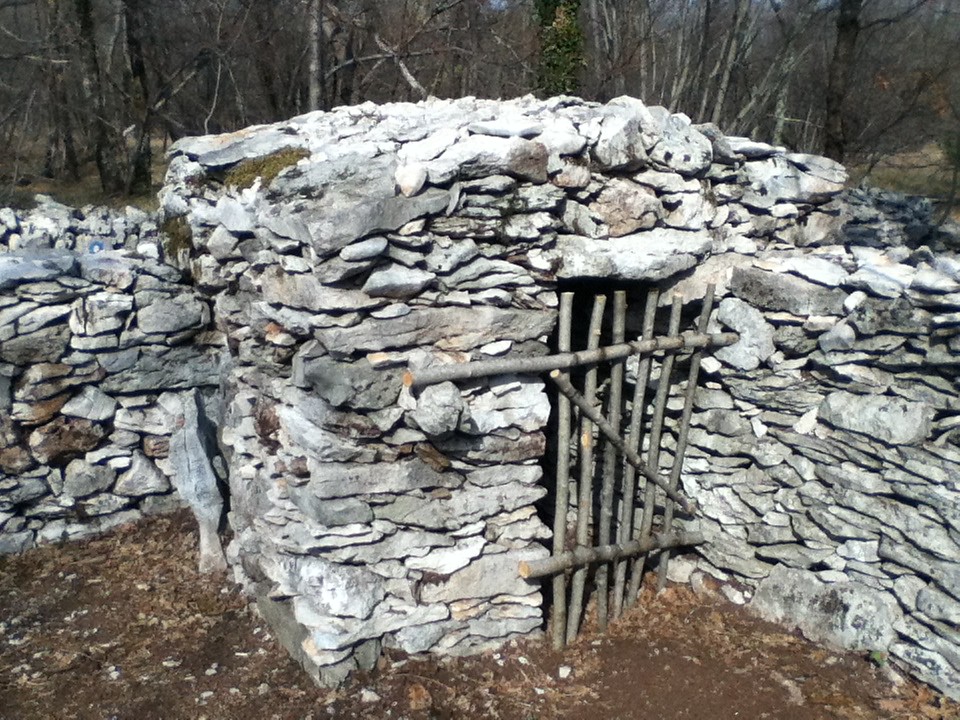The image features a small rock room nestled outdoors, created from numerous gray slate rocks meticulously stacked without the use of mortar. The structure includes a makeshift door crafted from sticks and tree branches, with one end inserted into a hole in the rock for support. The door comprises multiple horizontal limbs and appears to be lockable with a cross limb. This rock room, resembling a fortress or campsite shelter, stands about five feet tall and is part of a more extensive rock formation with a wall extending from its left side. Surrounding and behind the structure, more rocks are piled up in a similar fashion and hue, predominantly light gray with some appearing slightly mottled. The ground in the foreground is covered in brown dirt and mud, which seems to retain some moisture. In the background, barren trees without leaves frame the rock room, indicating a likely cold day in an outdoor woodland setting.